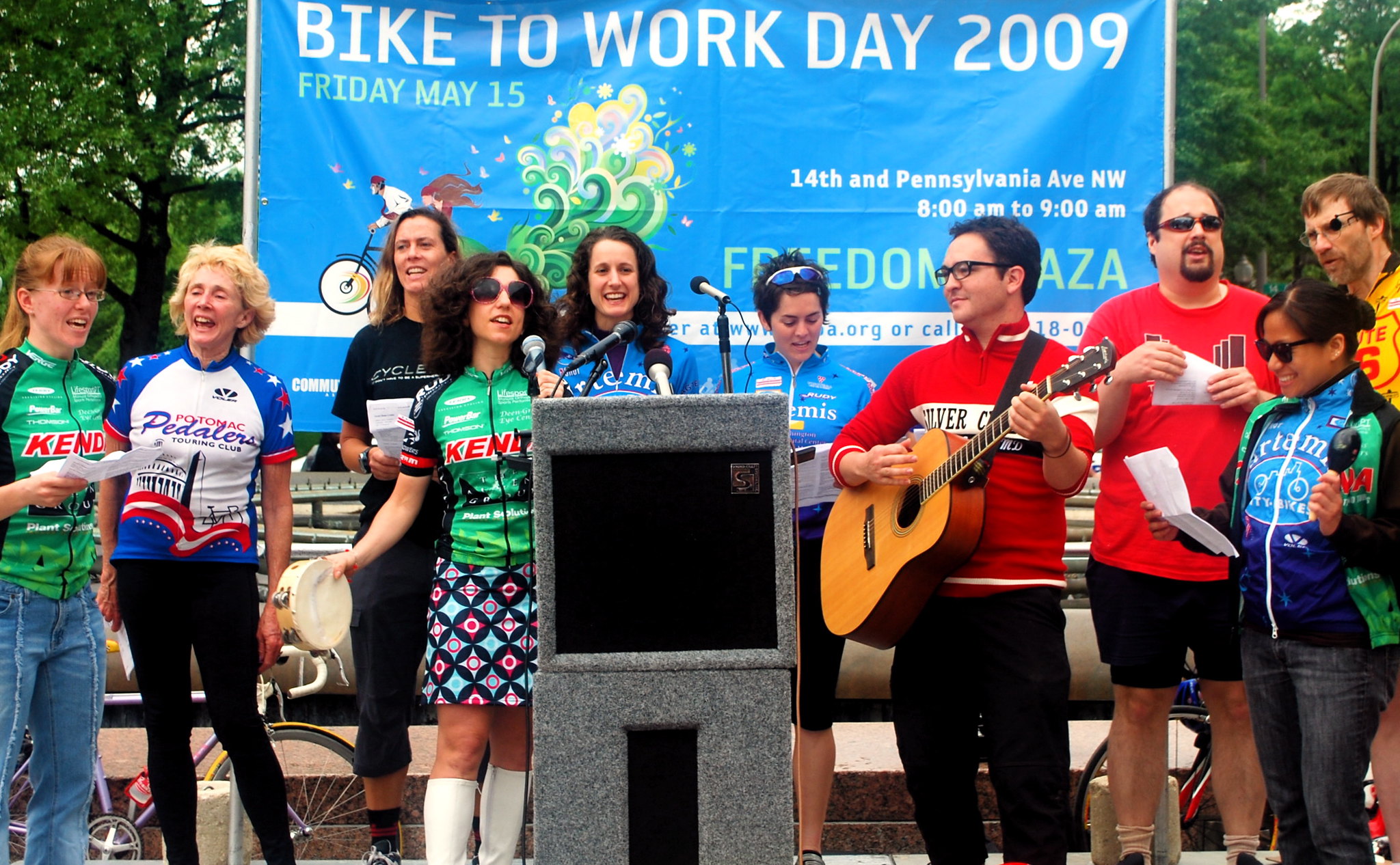In this vibrant outdoor scene at a park, an enthusiastic crowd dressed in active wear and bicycle jerseys gathers around a stage set for a special event. The backdrop is lush with greenery, indicating the park setting, while a prominent light blue banner with white lettering announces "Bike to Work Day 2009, Friday, May 15th, 14th and Pennsylvania Avenue NW, 8am to 9am, Freedom Plaza." 

On stage, a diverse group of performers engages the audience. A woman with long shaggy brown hair and round glasses, dressed in a bicycle shirt paired with a retro skirt featuring red and blue diamonds and white circles, holds a tambourine and a microphone. Beside her is a man in a red bicycle jersey strumming an acoustic guitar. Another woman, accompanied by shakers, adds to the rhythm, creating a lively and communal atmosphere.

In front of the performers stands a large gray podium adorned with two microphones, signifying the importance of the event and perhaps hinting at upcoming speeches or announcements. Surrounding the stage, many attendees hold white pieces of paper, suggesting they might join in a song or chant, ready to celebrate and commemorate the significance of cycling to work. The ambiance is filled with excitement and camaraderie as everyone prepares to enjoy this spirited event.